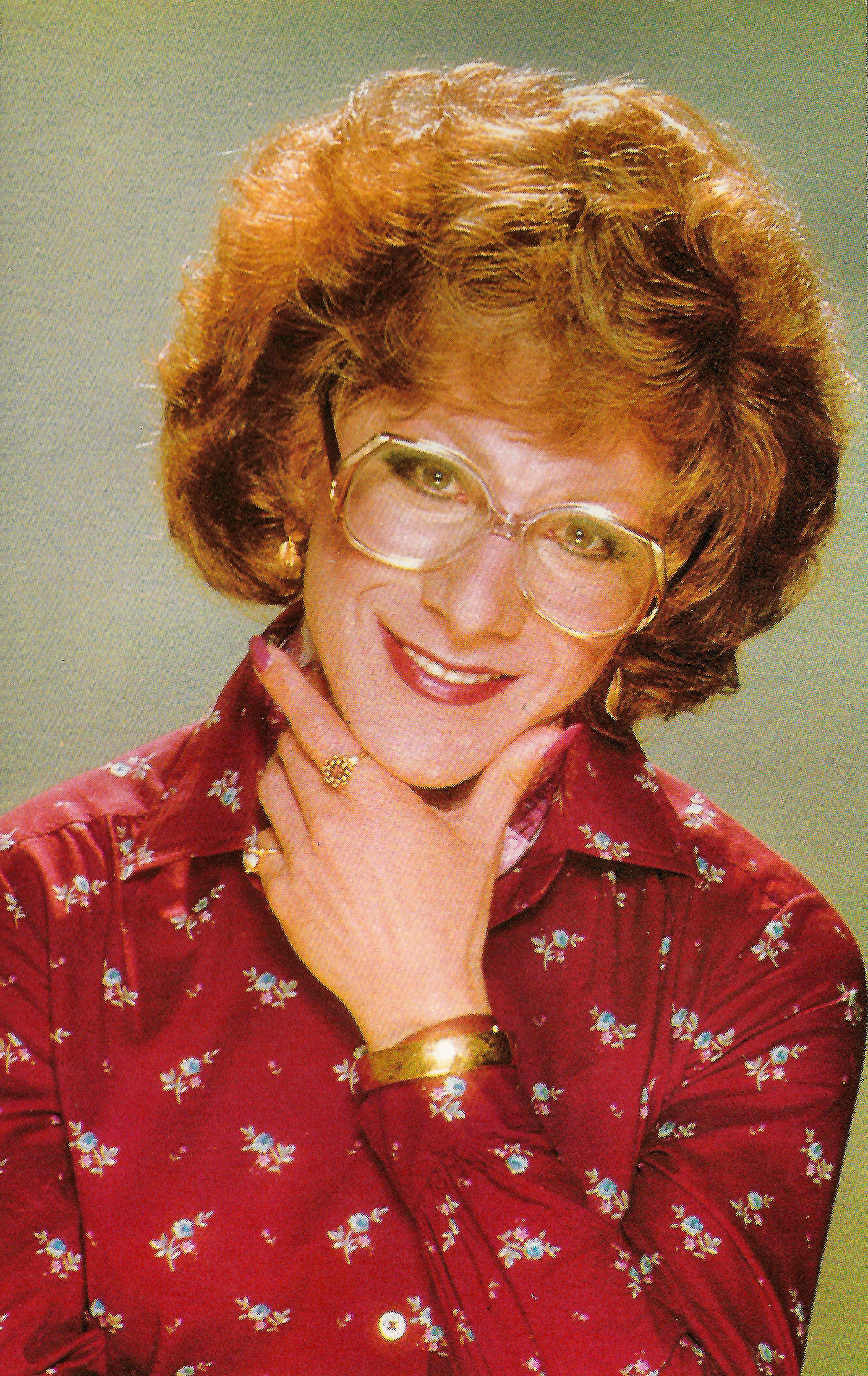In this 1980s-inspired portrait, a woman is captured from the chest up, exuding classic retro charm. She is dressed in a vibrant red satin shirt adorned with a delicate pattern of blue flowers. The shirt's glossy finish and collared design add a touch of elegance. Draped around her wrist is a gold bracelet, complementing her overall look.

Striking a thoughtful pose with her hand gently resting on her chin, she radiates confidence and grace. Her nails are painted a soft pink, adding a subtle but feminine detail. She wears distinctive large, circular glasses with clear frames, which enhances her sophisticated, vintage appearance.

Her voluminous, medium-length hair is styled into a helmet-like shape, characterized by its bouncy curls, contributing to the portrait's nostalgic 80s vibe. Her makeup is elegantly done: a bold red lipstick, understated eye makeup, and gold earrings that catch the light perfectly. 

With a gentle smile on her face, she engages warmly with the camera. The simplicity of the plain white studio background, accented with a hint of green, ensures that she remains the focal point of this evocative and stylish image.